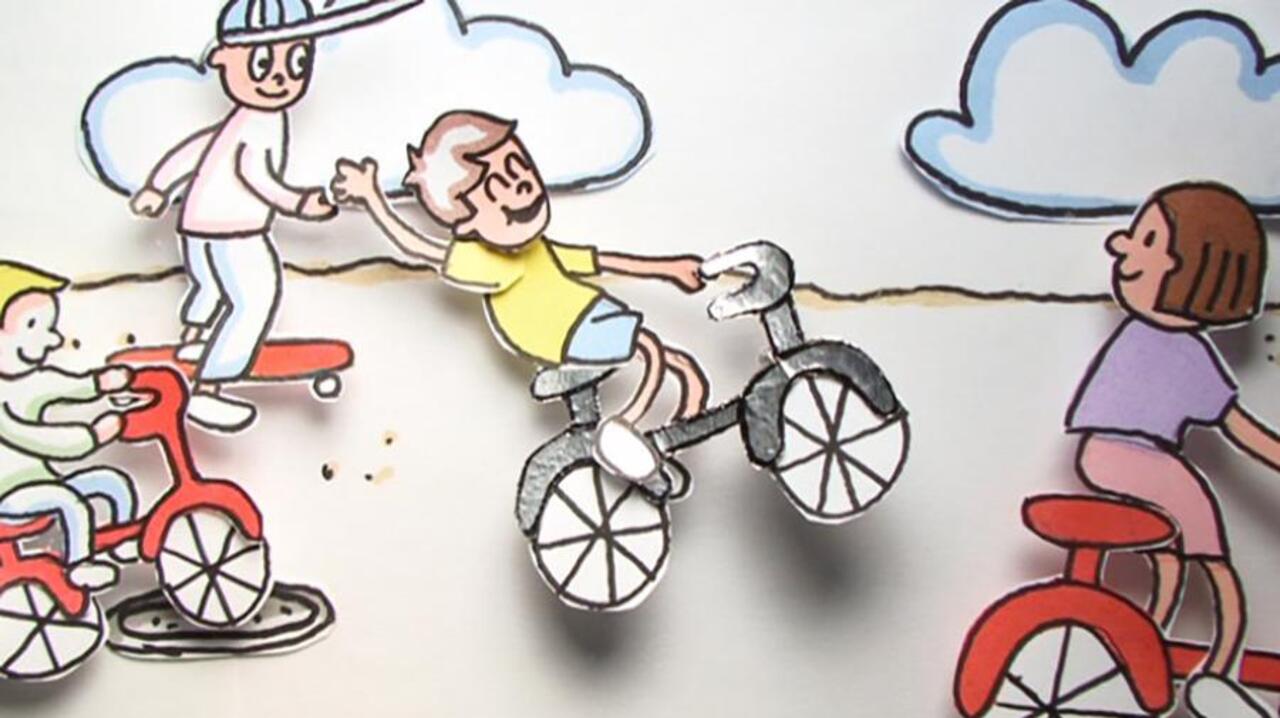The image depicts a three-dimensional cartoon scene made from colored paper cutouts, showcasing a group of children enjoying outdoor activities on a cream-colored surface. Positioned centrally, there's a young boy with brown hair, donning a yellow shirt and blue shorts, energetically riding a black bicycle with one hand raised as if in mid-celebration. To his right, a girl with shoulder-length brown hair, wearing a pink t-shirt and yellow and pink shorts, is seen riding a red bicycle, smiling at the boy. Above and to the left of the central boy is another boy with blonde hair, dressed in a light blue long-sleeve shirt and light blue pants, riding a red bike. In the rear and slightly behind the central figures, a boy clad in a white shirt and light blue pants, sporting a large blue baseball cap, is riding a red skateboard. The background features a simplistic landscape with two clouds and a white line marking the horizon, adding depth to the playful scene.